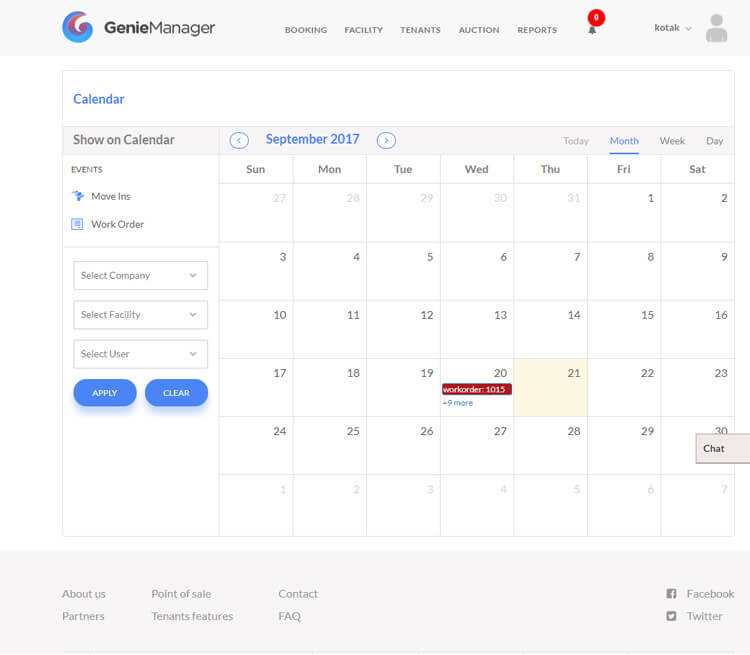This image is a detailed screenshot of the website "GenieManager," a platform designed for comprehensive calendar and task management, suitable for both personal and business use. The interface prominently features a large calendar in the center, set to September 2017. The clean, white background of the site accentuates its organized layout. 

In the upper left, the word "GenieManager" is displayed alongside the company’s logo—a stylized 'G' in blue and purple hues. The top center of the screen includes navigational links labeled "Booking," "Facility," "Tenants," "Auction," and "Reports," which direct users to various functionalities within the platform.

Dominating the central part of the screen is the calendar view, housed within a white box with a delicate gray outline. The heading "Calendar" appears in blue text at the top left of this section. The month view of September 2017 is mostly unoccupied, except for September 20th, which stands out with a red box labeled "Work Order 1015." This box also indicates that there are "plus 9 more" tasks scheduled for the day, suggesting a total of ten entries.

To the left of the calendar, there is a sidebar featuring options to add various types of events, such as move-ins or work orders. Users can also select the relevant company, facility, or user for each entry, indicating that this tool is tailored for property or apartment complex management.

At the bottom of the page, links to "About Us," "Partners," "FAQ," and other sections provide additional resources and information about GenieManager. In the bottom right corner, direct links to GenieManager's Facebook and Twitter accounts are displayed, encouraging users to connect via social media.